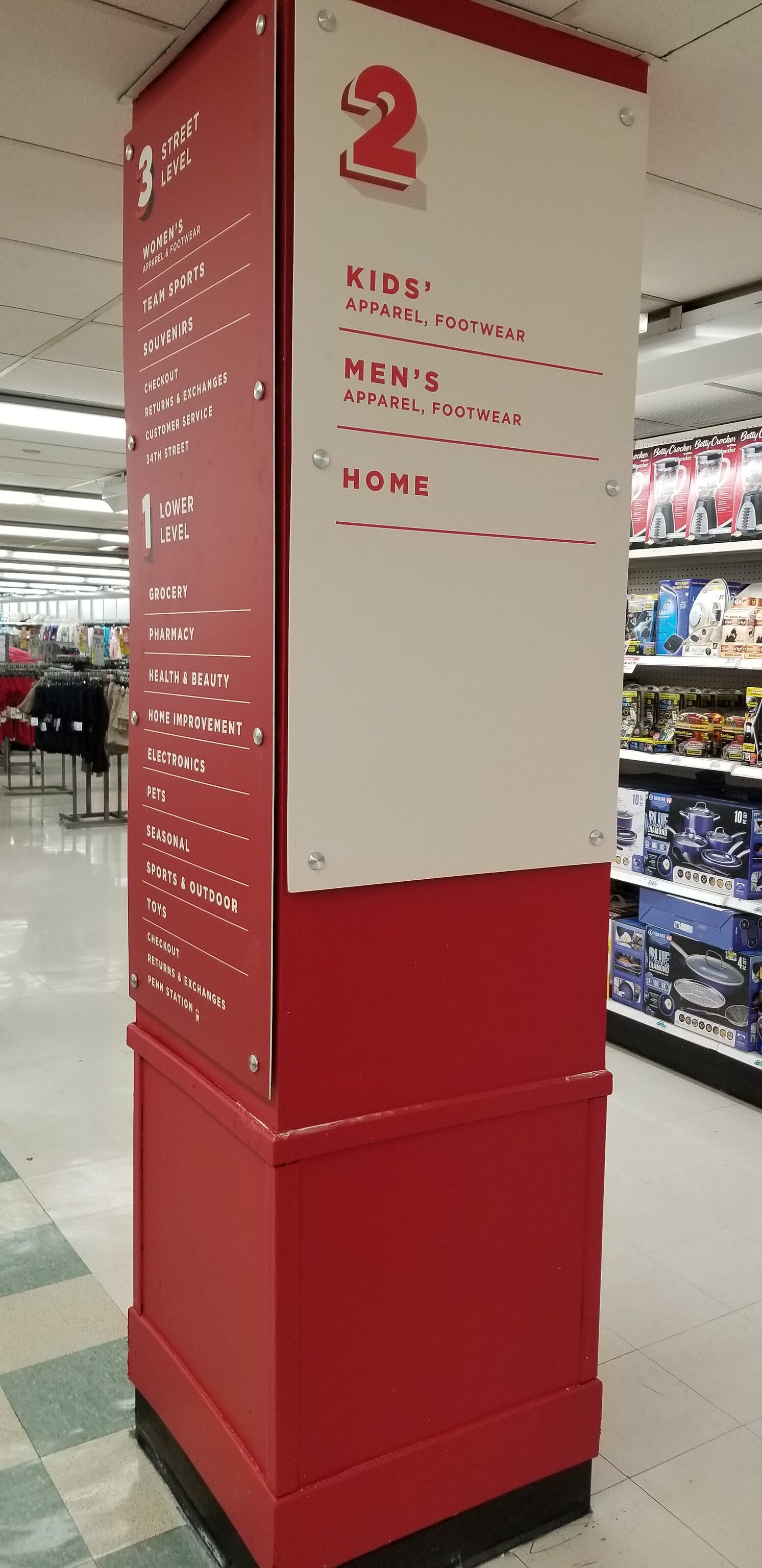The image depicts a first-person perspective inside a large department store or big box store, featuring a prominent, square-shaped red pillar situated in the middle of an aisle. The pillar stands on a shiny, linoleum-tiled floor that transitions from predominantly white tiles to a gray and white checkered pattern on the left side. The pillar, which functions as a navigational aid, displays directional signage on two visible faces. 

On the left face, a red sign lists various store sections by floor levels, starting with "Three Street Level" including "Women's" and "Team Sports," followed by "One Lower Level" indicating "Grocery," "Pharmacy," and "Health and Beauty." On the right face, a white sign displays a large number "2" at the top, with the following sections listed underneath: "Kids' Apparel, Footwear," "Men's Apparel, Footwear," and "Home." The photo captures the scene from an angle that showcases both signs, with merchandise neatly arranged on shelves and some clothing racks visible in the background, all under well-lit conditions.